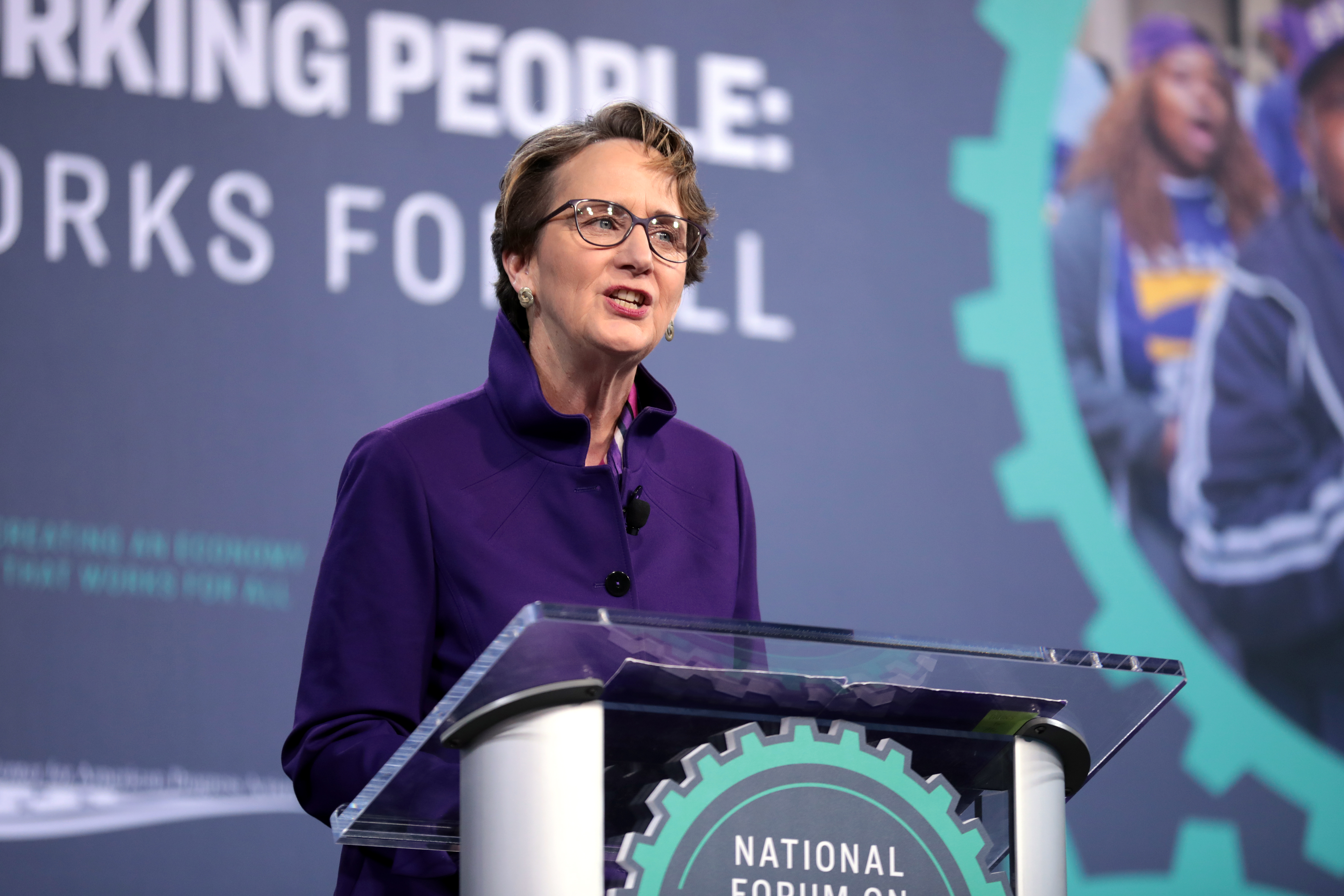The photograph captures an older woman with short light brown hair, wearing dark-rimmed glasses and two round earrings, standing on a stage behind a lectern. She is speaking at an event, her mouth open mid-sentence as she looks intently to the side. She is dressed in a long-sleeve purple shirt, though another description mentions a blue coat with large black buttons and a high collar, suggesting possible color variation or layers. A lapel microphone is attached to her collar.

In the background, there is a large, slightly blurry image on a navy blue canvas. Prominent white letters form partial words: "king," "R-K-S," "F-O," and two "Ls," though the full context is cut off. To the left of this text is a mint-green cog-shaped semi-circle with an image of two people inside, partially obscured. The lectern she stands behind bears the word "national," though the rest of the text is not visible. The overall scene suggests a formal speaking engagement or conference.